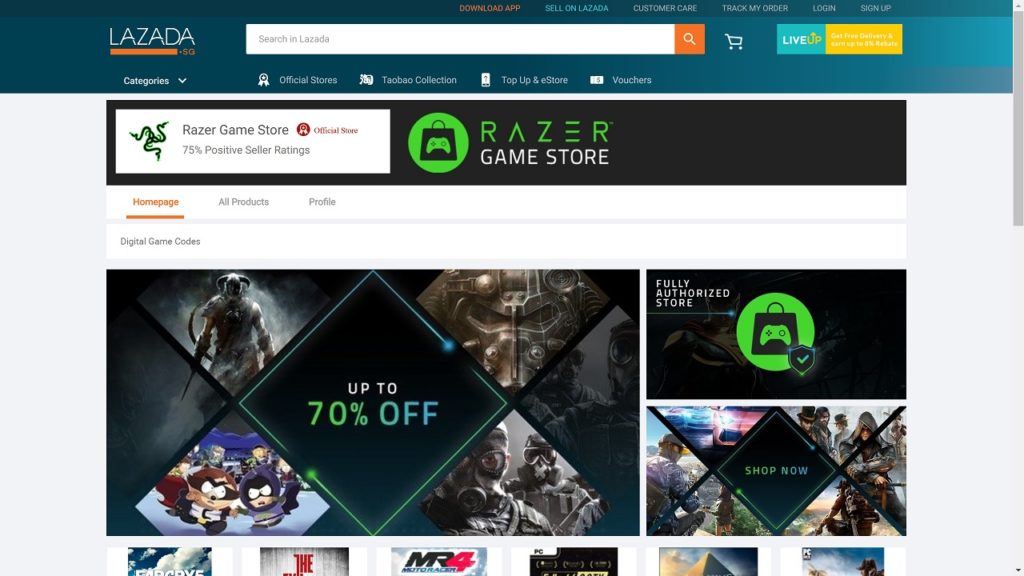The image showcases the homepage of the Lazada website. At the top left corner, the Lazada logo is distinctly visible, encased in a bluish-colored box. The brand name "Lazada" is prominently displayed in white font with a thick orange underline, followed by the abbreviation "SG" in orange font. To the right of the logo, there is a white search box with placeholder text that says "Search in Lazada," accompanied by an orange search button.

Above the search box, there is a horizontal menu featuring six options: "Download App," "Sell on Lazada," "Customer Care," "Track My Order," "Log In," and "Sign Up." Continuing to the right, a shopping cart icon is visible, followed by a blue and yellow box labeled "LiveUp," which offers delivery benefits and potential earnings, albeit the exact percentage is blurred and hard to read. Below this top section, additional navigation options are presented within the same bluish gradient box, including "Categories," "Official Stores," "Taobao Collection," "Top Up & E-Store," and "Vouchers."

The main content of the website is set against a grayish-white background. A prominent banner announces the "Razer Game Store," suggesting that the viewer has navigated to this specific store on the platform. The store's homepage features tabs for "All Products" and "Profile." A black banner within this section indicates that the Razer Game Store is an official store on Lazada, boasting a 75% positive seller rating. Additionally, there are options to explore "Digital Game Codes" and various product categories within the store.